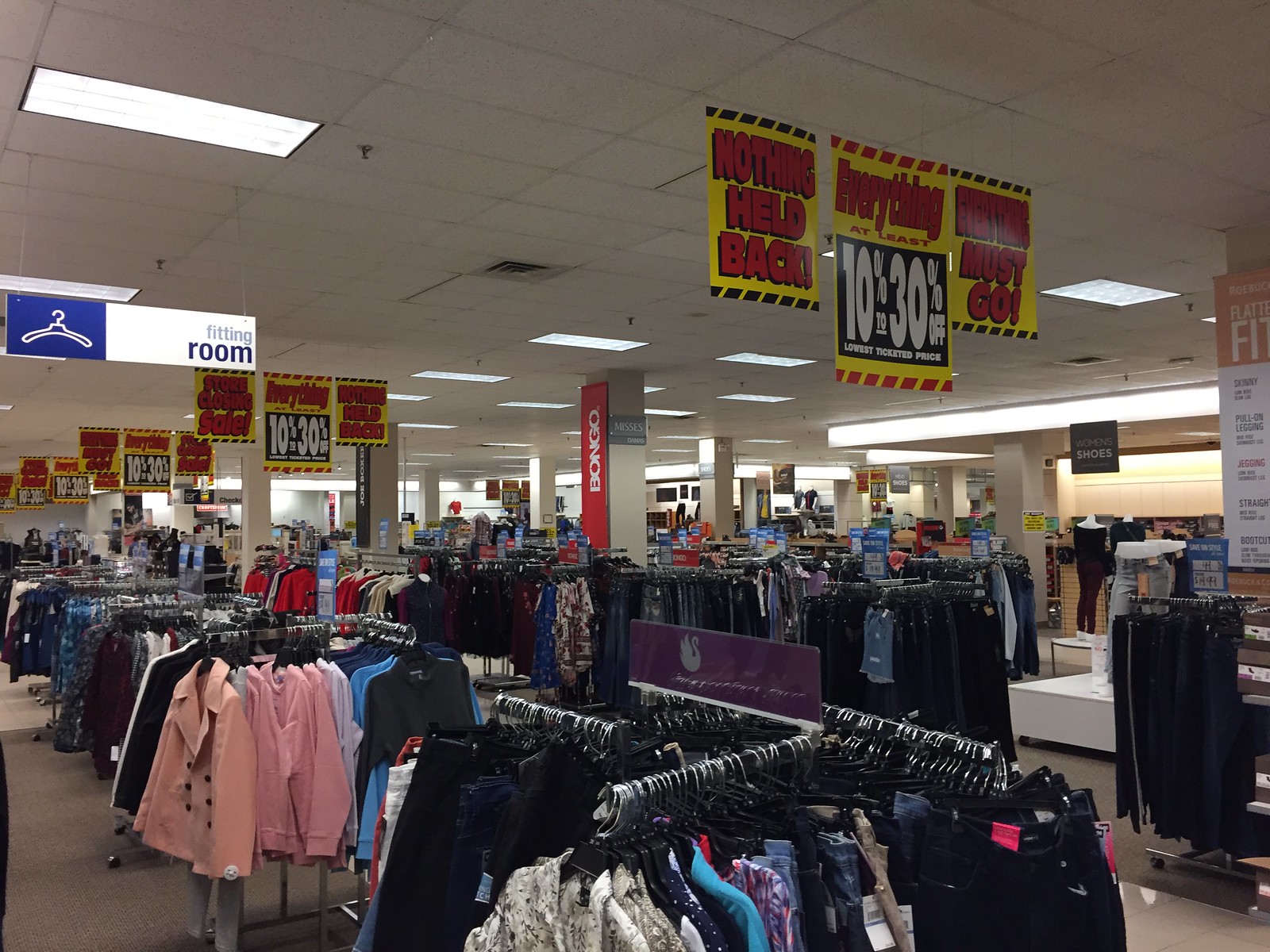The photograph captures the interior of a brightly-lit clothing store filled with numerous garment racks stretching into the distance. The ceiling, characterized by its white drop tiles suspended within a grey lattice structure, features multiple prominent signs that indicate a substantial sale event. Three yellow signs with bold red text hang in the foreground on the right side: one reads "Nothing Held Back," the next announces "Everything At Least 10% to 30% Off," and the third proclaims "Everything Must Go." These signs give the impression of a significant clearance sale, possibly suggesting the store is closing down.

To the left, towards the back of the store, a fitting room sign with a distinctive blue background catches the eye; it features a white coat hanger graphic on the left side and the words "Fitting Room" in bolder text on the right side of the rectangular sign. Amidst the racks of clothing, several mannequins display outfits like leggings and black tops, and a sign on a pillar says "BONGO" in red letters. The aisles are densely packed with modern and possibly vintage garments, including jackets that resemble styles from the 1980s, complete with shoulder pads. The overall atmosphere is reminiscent of a large-scale, possibly final, clearance reminiscent of closing down sales historically associated with stores like Kmart.